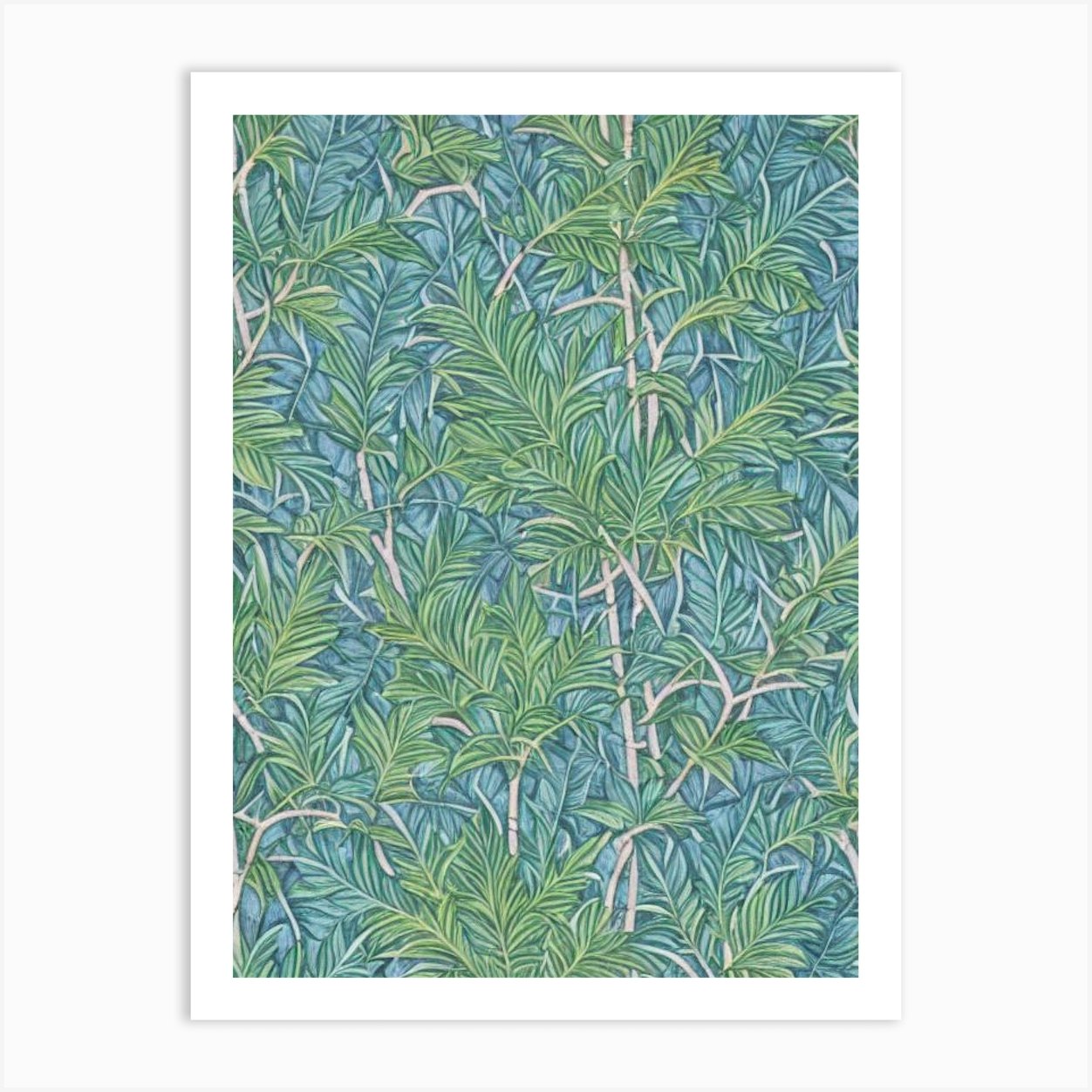The image features a vibrant, detailed painting of dense tropical trees set against a white background. The composition showcases a variety of trees and branches, focusing primarily on the lush foliage. The leaves are depicted in two distinct layers: the background layer consists of teal and turquoise blue leaves, while the overlaying layer features an array of green hues, including light green, dark green, and lime green. The slender and fan-like leaves resemble tropical vegetation, with some tree trunks visible that bear a resemblance to bamboo. The branches are painted white, adding contrast to the rich, green foliage, creating a striking visual. This artwork could also serve as a wallpaper, greeting card, wrapping paper, or even a computer background, given its seamless, all-encompassing pattern of trees and leaves intricately woven together.